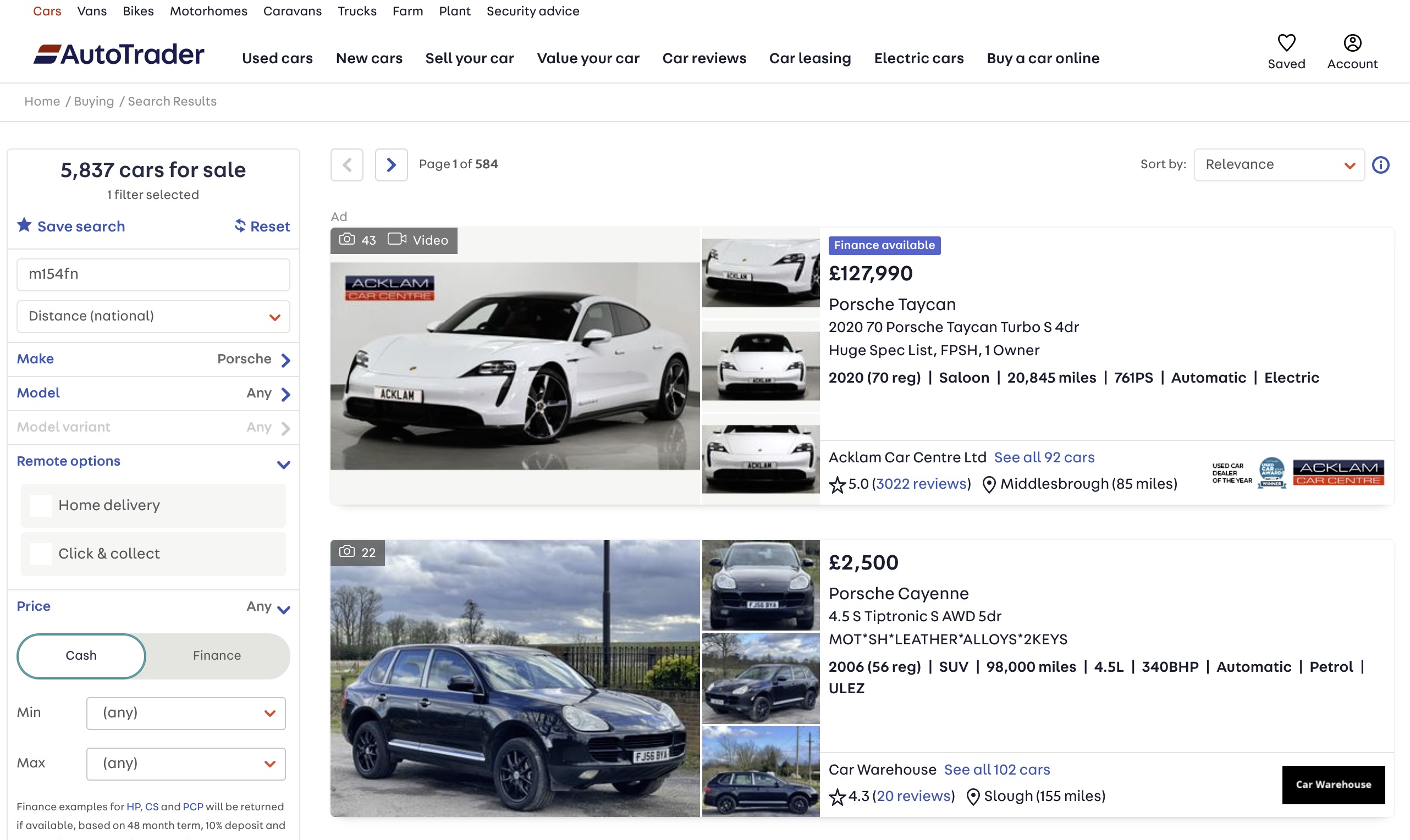A screenshot of an Auto Trader website with a white background and black text features prominently displayed at the top. The Auto Trader logo is situated in the top left corner, accompanied by a blue and red horizontal line. The main navigation bar includes various options such as "Cars" (highlighted in red), "Vans," "Bikes," "Motorhomes," "Caravans," "Trucks," "Farm," "Plant," "Security Advice," "Used Cars," "New Cars," "Sell Your Car," "Value Your Car," "Car Reviews," "Car Leasing," "Electric Cars," and "Buy a Car Online."

There are currently 5,837 cars listed for sale. Users can save their search and filter results based on distance, make, model, variant, delivery options, payment methods (cash and finance), as well as minimum and maximum price ranges.

In the center of the screen are pictures of two cars. The first is a flashy silver sports car—a 2020 Porsche Taycan Turbo S 4DR—with a price tag of £127,990. Key details include 20,845 miles, FPSH, one owner, automatic electric transmission, and a massive spec list. It is sold by Acklam Car Centre Limited, which has 92 cars listed for sale and maintains a 5.0-star rating. The dealership is located 85 miles away from the searcher in Middlesbrough.

Below the sports car is a small, dark blue (almost black) hatchback, priced at £2,500. Despite being listed as a Porsche Taycan, its appearance and price suggest otherwise. It is described as a 4.5 S Tiptronic S AWD 5DR with 98,000 miles, automatic petrol transmission, low MOT, SH, leather upholstery, alloy wheels, and two keys, making it a 1,650 Reg SUV in Slough, 155 miles away from the searcher. It is offered by Car Warehouse, which has 102 cars for sale and a 4.3-star rating.